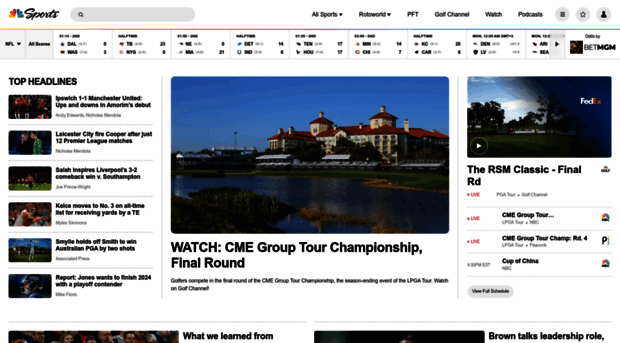The image is a screenshot from a sports website, likely affiliated with ABC Sports, featuring a prominent emblem that resembles turkey feathers spread out at the top with the word "SPORTS" emblazoned across it. At the very top of the screen lies a gray search bar, flanked by various navigational links such as "All Sports," "Roto World," "PFT," "Golf Channel," "Watch," and "Podcast." Furthermore, the uppermost section of the image displays live baseball scores, indicating it is the top of the eighth inning for several games, alongside the date "June 23rd."

Towards the top right, an eye-catching blue circle with a white exclamation point houses a prompt that reads, "How to watch Noah Lyles and other track and field stars in the men's 100-meter at U.S. Olympics Trials on NBC and Peacock." Below this section lies clickable content that includes a link titled "six hours of the Glen" and another for watching the "KPMG Women's PGA Championship Final Round."

On the right-hand side of the image, the "Top Headlines" section is visible, showcasing six smaller pictures, each linked to different articles, offering a quick visual navigation to the most recent sports news and updates.